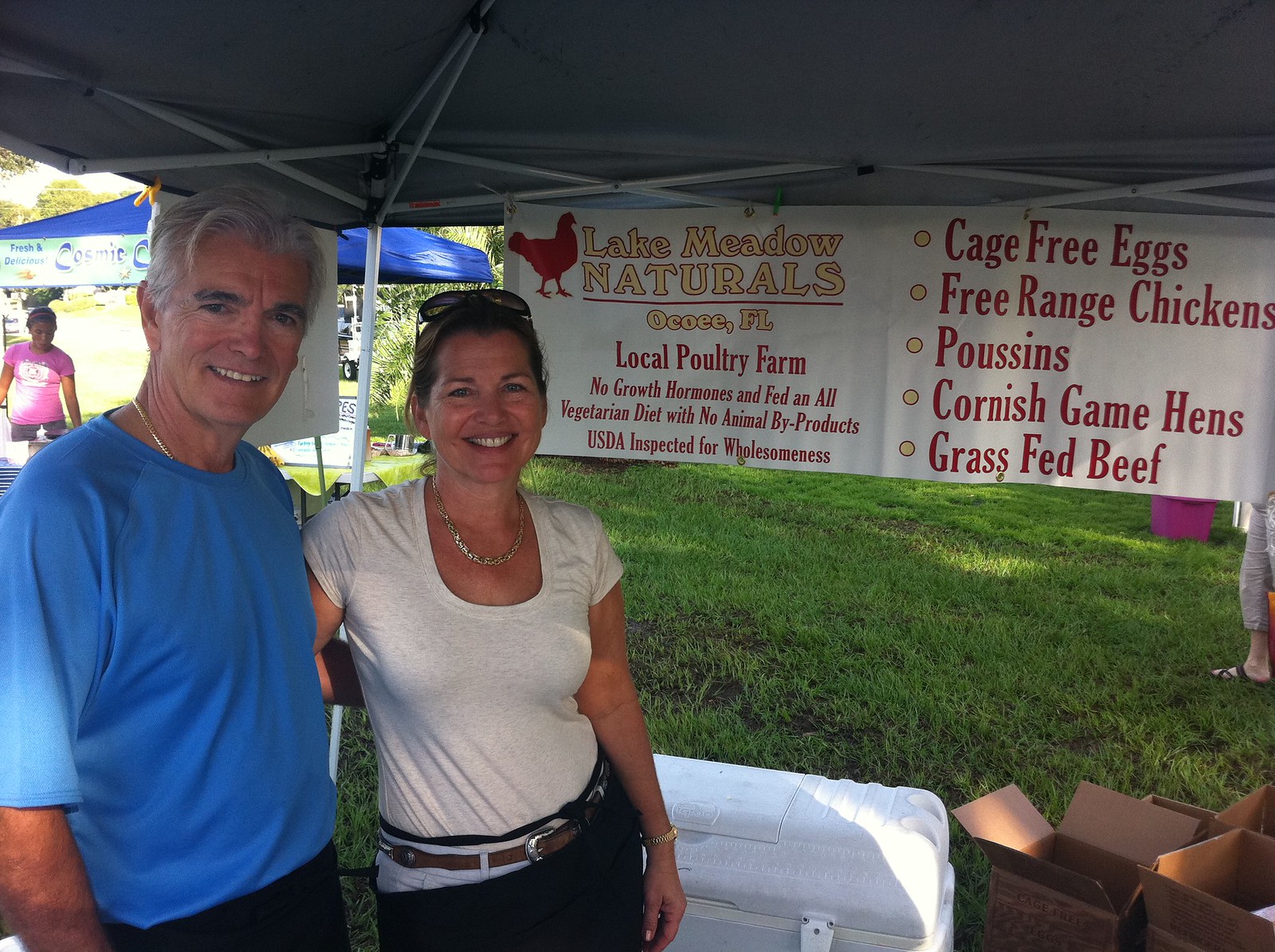In the foreground of this outdoor photograph, a couple is standing on the left side, arm-in-arm and smiling under a gray canopy. The man, who appears middle-aged with gray hair and fair skin, is wearing a light blue t-shirt, black pants, and a gold necklace that peeks out from under his shirt. He has dark eyebrows and a clean-shaven face. Beside him, a younger fair-skinned woman with dark hair pulled back and sunglasses resting on her head is dressed in a white t-shirt and dark pants, also wearing a necklace. Both are exuding happiness as they pose together. Behind them, a white cooler and a couple of open cardboard boxes can be seen on the grass.

The background features a large banner with prominent red and yellow text. The banner, hung under the blue canopy where another woman in a pink t-shirt stands in the far back corner, showcases a red chicken logo and reads "Lake Meadow Naturals" followed by "Ocala, Florida" in bold red letters. Below this, it claims "Local Poultry Farm" and lists "Cage-Free Eggs, Free-Range Chickens, Poussins, Cornish Game Hens, and Grass-Fed Beef." The scene clearly represents a vibrant and friendly market or event, with the couple enjoying their time amidst the stalls.